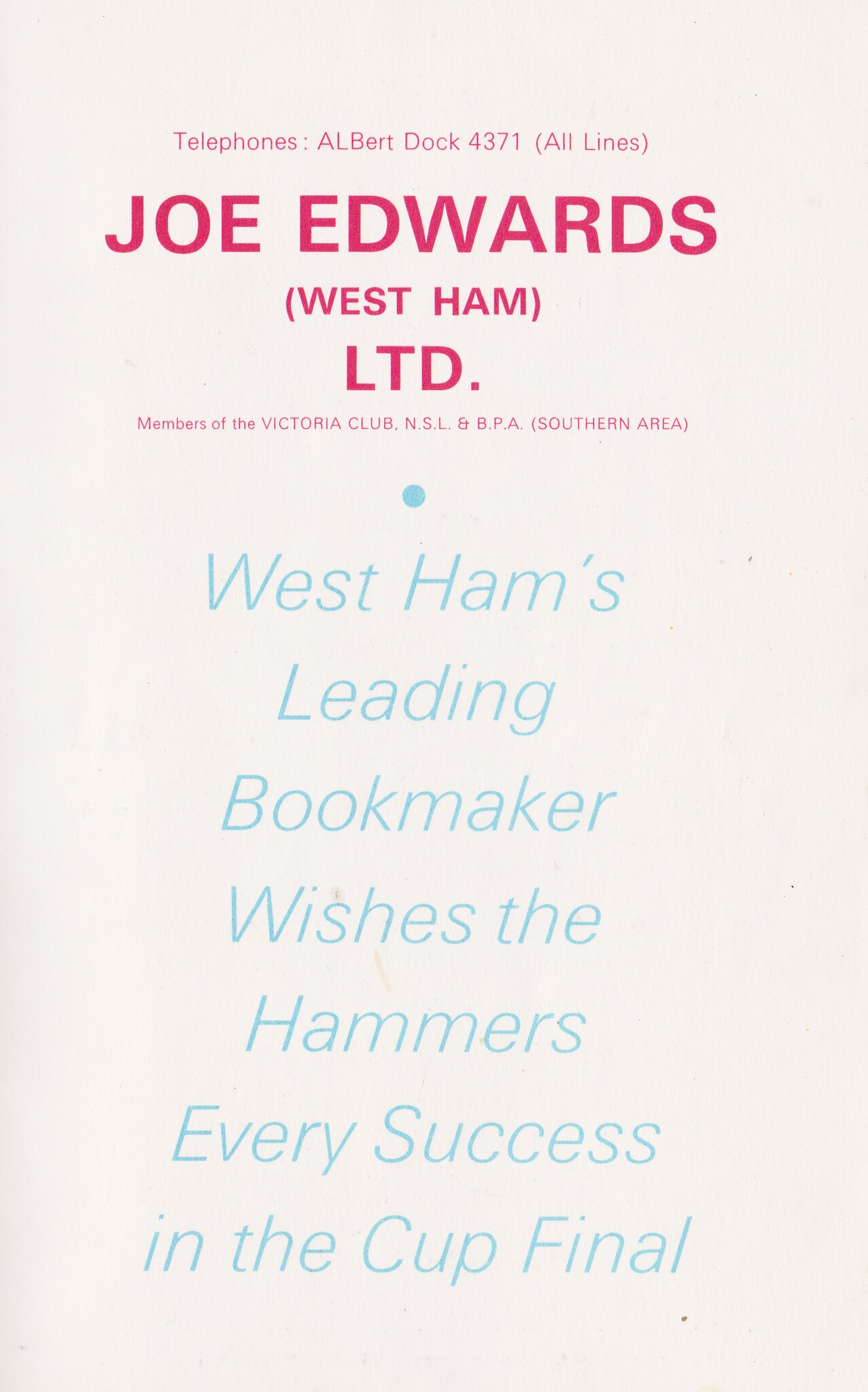The image shows a sign with a white cream background. At the top in small, bold red letters, it reads: "Telephones, Albert, Doc, 4371, in parentheses, All Lines." Beneath that, in larger bold red letters, it says "Joe Edwards". Following in red, it mentions "West Ham" in parentheses, then "LTD." Below it, the text continues, stating "Members of the Victoria Club, NSL, and BPA, Southern Area". There’s a small blue dot below this section. Underneath the dot, in thin blue letters spread across seven lines, it reads: "West Ham's leading bookmaker wishes the Hammers every success in the cup final." The varied font styles and colors distinguish different sections of the sign, conveying both informational and promotional details without any people in the photo.